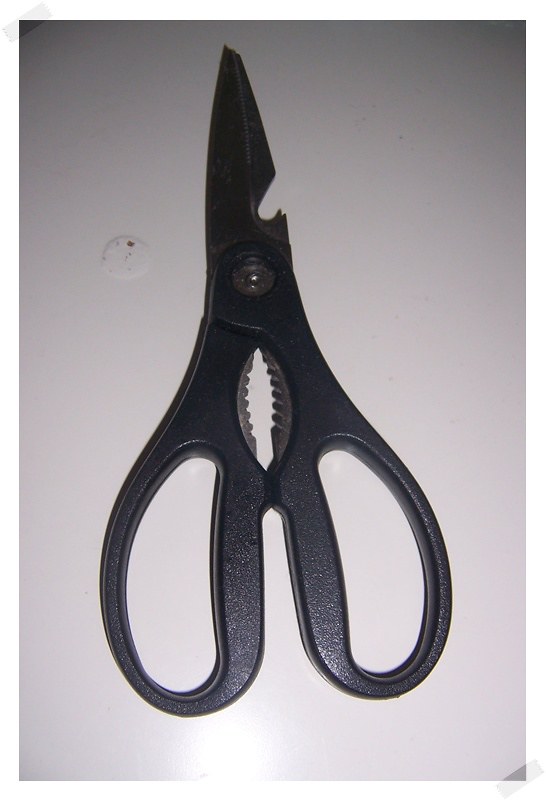This image features a pair of black-handled scissors prominently displayed on an off-white to grayish-white gradient background. The scissors are oriented vertically, with the sharp ends pointing slightly to the left of vertical, akin to 11:30 on a clock. The background is brighter at the bottom center, where it reveals a glare that diminishes as the gradient darkens towards the top of the image. Midway down the blades, there is a small notch shaped like a half-heart or bottle opener, adding a distinct detail to their design. The handles are black plastic, and above the pivot point between them, there is a football-shaped opening with a metal insert featuring toothed edges. To the left of the blades, an imperfection in the surface, possibly a paint drip, introduces an additional element to the overall composition. A tiny piece of tape is noticeable in the bottom right-hand corner, adding another layer of texture to the scene.